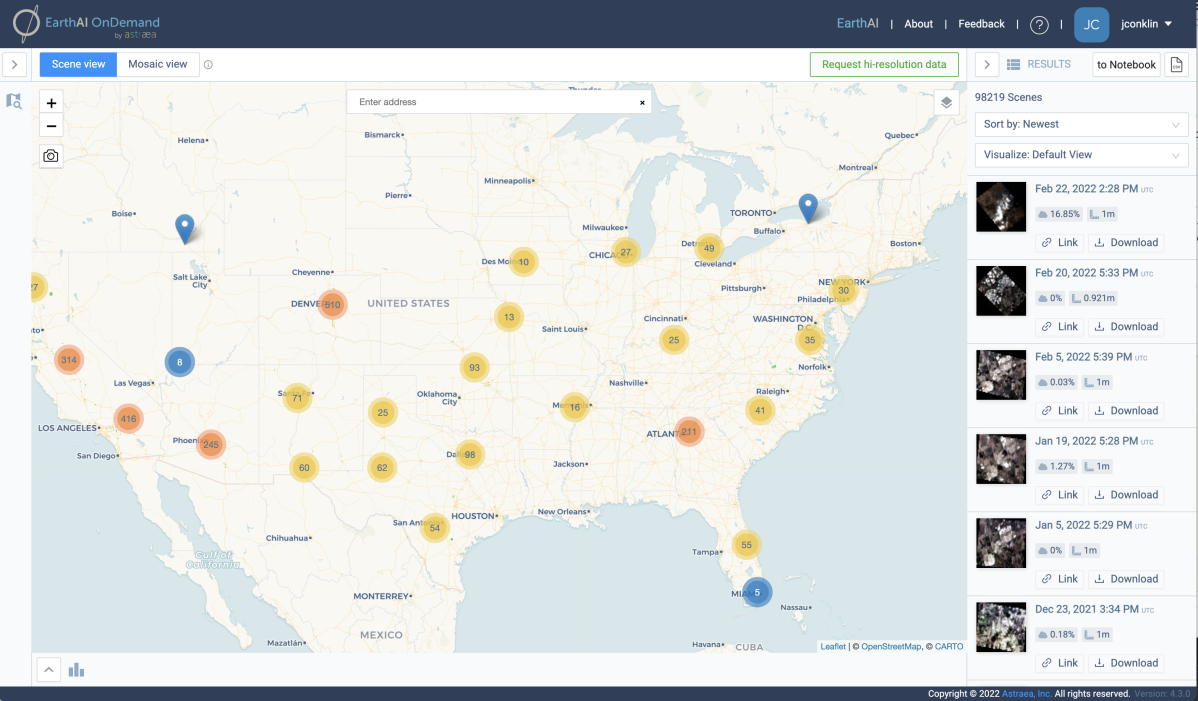**Image Description: Detailed Overview of the "Earth AI On Demand" Website Interface**

The screenshot displays an interface of a website featuring a map functionality. 

At the very top, a dark blue navigation bar spans across the width of the screen. On the left side of this bar, there's a distinctive logo resembling the planet Saturn with a ring encircling it. To the right of this logo, the text “Earth AI on demand” is displayed, where the words “Earth” and “on demand” are in blue, while “AI” is in white. Beneath this text, there's some very small, thin text, which is not legible.

On the right side of the navigation bar, the menu options appear in a horizontal sequence separated by vertical lines:
- “Earth AI”
- “About”
- “Feedback”
- A question mark inside a circle
- A blue rounded-corner square with lighter blue inside, containing the white initials “JC”
- An adjacent drop-down menu, possibly showing the username, starting with "J"

Below this header, the main content area is divided into two primary sections: the map on the left and a sidebar on the right.

**Left Section: Map Interface**
- The top portion has several buttons:
  - A square with a greater than symbol “>”
  - A blue button with unreadable text
  - A button labeled “Screen View”
  - A button with a white background labeled “Mosaic View”
  - A button with a green outline marked “Request High-Resolution Data”
  - A greater than symbol followed by the text “Results to Notebook”
  - A page icon
  
- The map itself features oceanic areas in blue and displays a detailed line map of the United States. Various colored circles (yellow, red, and blue) are scattered across the map, each likely indicating different data points. 
  - Approximately:
    - 10-20 yellow circles
    - 5 red circles
    - 2 blue circles
  - The map also highlights major cities and states, and includes parts of Canada and Mexico. Two location markers are visible.

**Right Section: Sidebar**
- At the top, the number “98,219 scenes” is displayed.
- Below this, there is a drop-down menu labeled “Sort by newest”.
- Another drop-down menu labeled “Visualize: Default View” follows.
- Below these menus, six rows of results are presented on a light blue background:
  - Each row includes:
    - A square thumbnail on the left, showcasing a dark image with some white elements (e.g., “February 22, 2022, 2:28 p.m.”)
    - Title text to the right of the thumbnail
    - Badges indicating details like “16%” and 1m with an “L” icon
    - Two buttons labeled “Link” and “Download”

Overall, the interface is structured to provide a comprehensive and interactive experience, with the map allowing users to view and interact with various data points, and the sidebar offering detailed insights and actions related to the selected scenes.